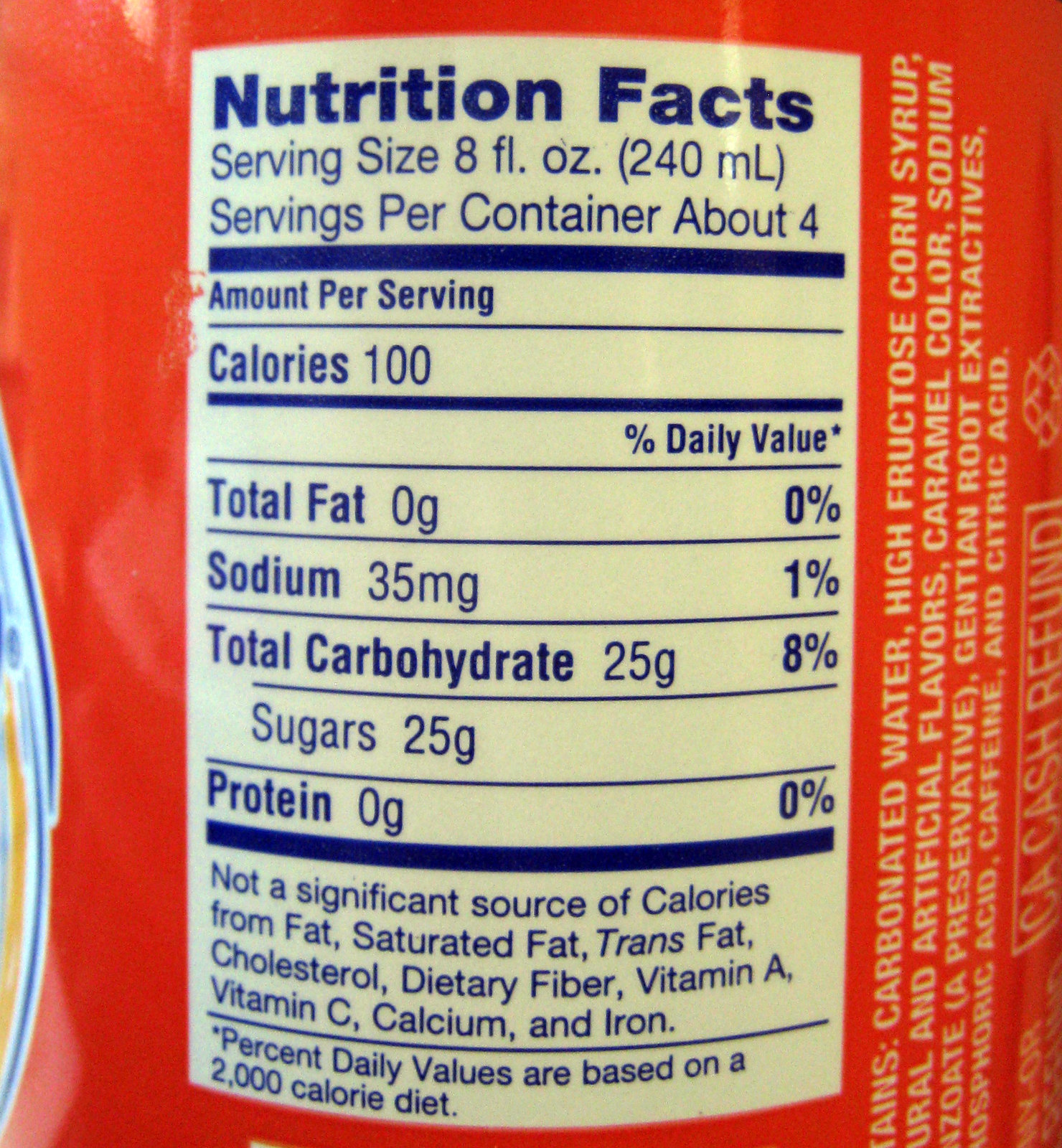The image captures the nutrition facts label on the side of a red food package, likely a soda bottle. The nutrition information is presented in a white box with navy blue text. The rounded label prominently displays “Nutrition Facts” at the top, followed by specifics: a serving size of 8 fluid ounces (240 milliliters), with 4 servings per container. Each serving provides 100 calories, 0 grams of total fat, 35 milligrams of sodium (1% DV), 25 grams of total carbohydrates (8% DV), all of which are sugars, and 0 grams of protein. The label also notes that the product is not a significant source of calories from fat, saturated fat, trans fat, cholesterol, dietary fiber, vitamin A, vitamin C, calcium, and iron. Percent daily values are based on a 2,000-calorie diet. Adjacent to the nutrition box, the ingredients list includes carbonated water, high fructose corn syrup, and artificial flavors. To the right, slightly off-screen, logos for CA cash refund and recycling can be seen, above circular patterns in blue, white, and yellow.